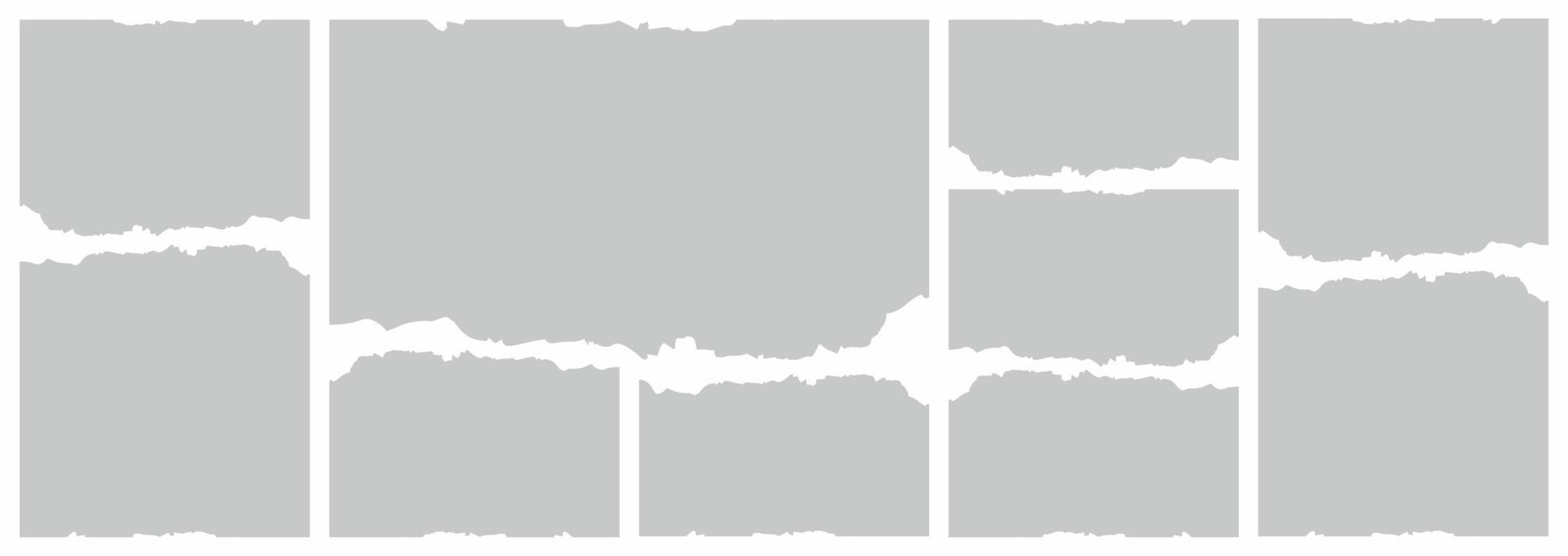The image depicts a minimalist piece of abstract art characterized by a horizontally rectangular layout. This artwork comprises ten individual gray shapes, which are either rectangular or square in form. Each shape is a uniform shade of pale gray, resembling a concrete color with the slightest hint of lavender. These shapes are arranged in rows and columns against a stark white background. The edges of each shape are notably jagged on the top and bottom, akin to torn paper, while the sides remain smooth. There is no text or additional colors present, emphasizing the simple yet striking composition of the gray shapes against the white backdrop. The overall effect is that of an enigmatic modern piece, possibly digital or painted, with a distinctly minimalist and concrete-like aesthetic.